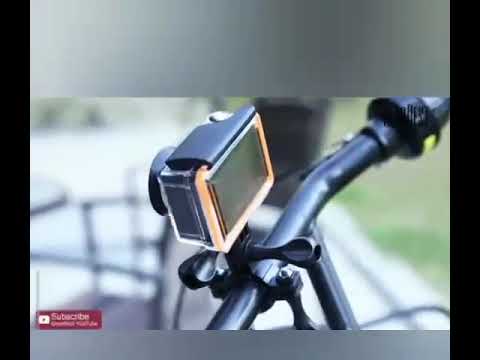This square photograph presents a detailed close-up of a bicycle handlebar situated in an outdoor setting. The composition is framed by solid gray horizontal borders at the top and bottom, with the top border being thicker, and black vertical borders on the left and right. Within these borders, the focus is on the right handlebar, which is black in color. Attached to the center of the handlebar is a small, square-shaped device, likely a camera or a GPS system, featuring a digital screen. The angle of the photo offers a partial, slightly blurry view of the right handlebar and part of the connecting bar, indicating a left-oriented perspective. In the bottom left corner, a YouTube subscribe icon is visible. The background reveals a concrete surface with some grass, enhancing the outdoor ambiance of the scene.